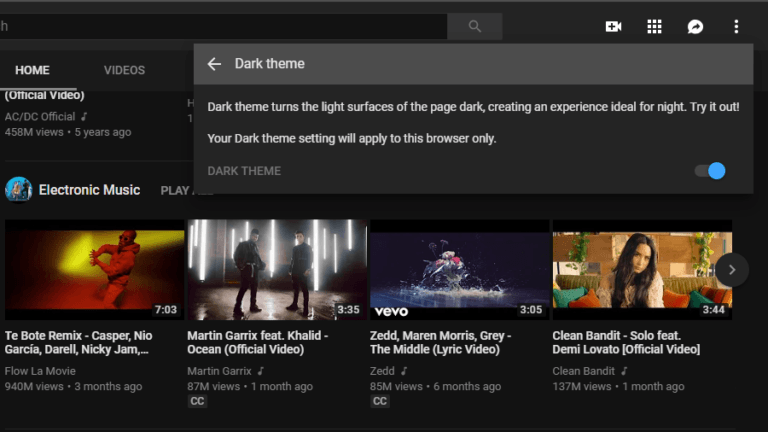The image showcases a user interface on a black background, primarily featuring a search bar at the top with a prominent search icon. The search bar is empty. Adjacent to it on the right are several icons: a square made up of small white dots, a white circle with an arrow in its center, and three vertical dots, likely representing a menu.

On the left sidebar, there are two options: "Home" and "Videos." "Home" is highlighted in white and underlined, while "Videos" is in gray. Below "Home," there is content listed with detailed descriptions:

1. **First Listing:**
   - Title: "Official Video, ACDC"
   - Channel: "ACDC Official"
   - Views: "458 million views"
   - Upload Time: "5 years ago"
   - Genre: "Electronic Music"
   - Thumbnail: An image of a musician with yellow and red shading.
   - Duration: "7 minutes and 3 seconds"

2. **Second Listing:**
   - Title: "Bote Remix"
   - Artists: "Casper, Neo, Garcia, Daryl, Nicky Jam"
   - Channel: "Flow La Movie"
   - Views: "940 million views"
   - Upload Time: "3 months ago"

3. **Third Listing:**
   - Title: "Ocean (Official Video)"
   - Artists: "Martin Garrix featuring Khalid"
   - Views: "87 million views"
   - Upload Time: "One month ago"
   - Duration: "3 minutes and 35 seconds"
   - Captions available: "CC"

4. **Fourth Listing:**
   - Title: "The Middle (Lyric Video)"
   - Artists: "Zedd, Maren Morris, Grey"
   - Views: "85 million views"
   - Upload Time: "6 months ago"
   - Duration: "3 minutes and 5 seconds"
   - Captions available: "CC"

5. **Fifth Listing:**
   - Title: "Solo (Official Video)"
   - Artists: "Clean Bandit featuring Demi Lovato"
   - Views: "137 million views"
   - Upload Time: "One month ago"
   - Thumbnail: Demi Lovato in a room filled with pillows
   - Duration: "3 minutes and 44 seconds"

At the top of these listings, a banner has popped up, announcing the "Dark Theme." The banner has a dark gray background with text in white explaining that the dark theme turns the light surfaces of the page dark, ideal for nighttime use. It further mentions that the dark theme setting will apply only to the current browser. There is a toggle button on the right side of the banner, which is blue indicating that the dark theme is currently activated.